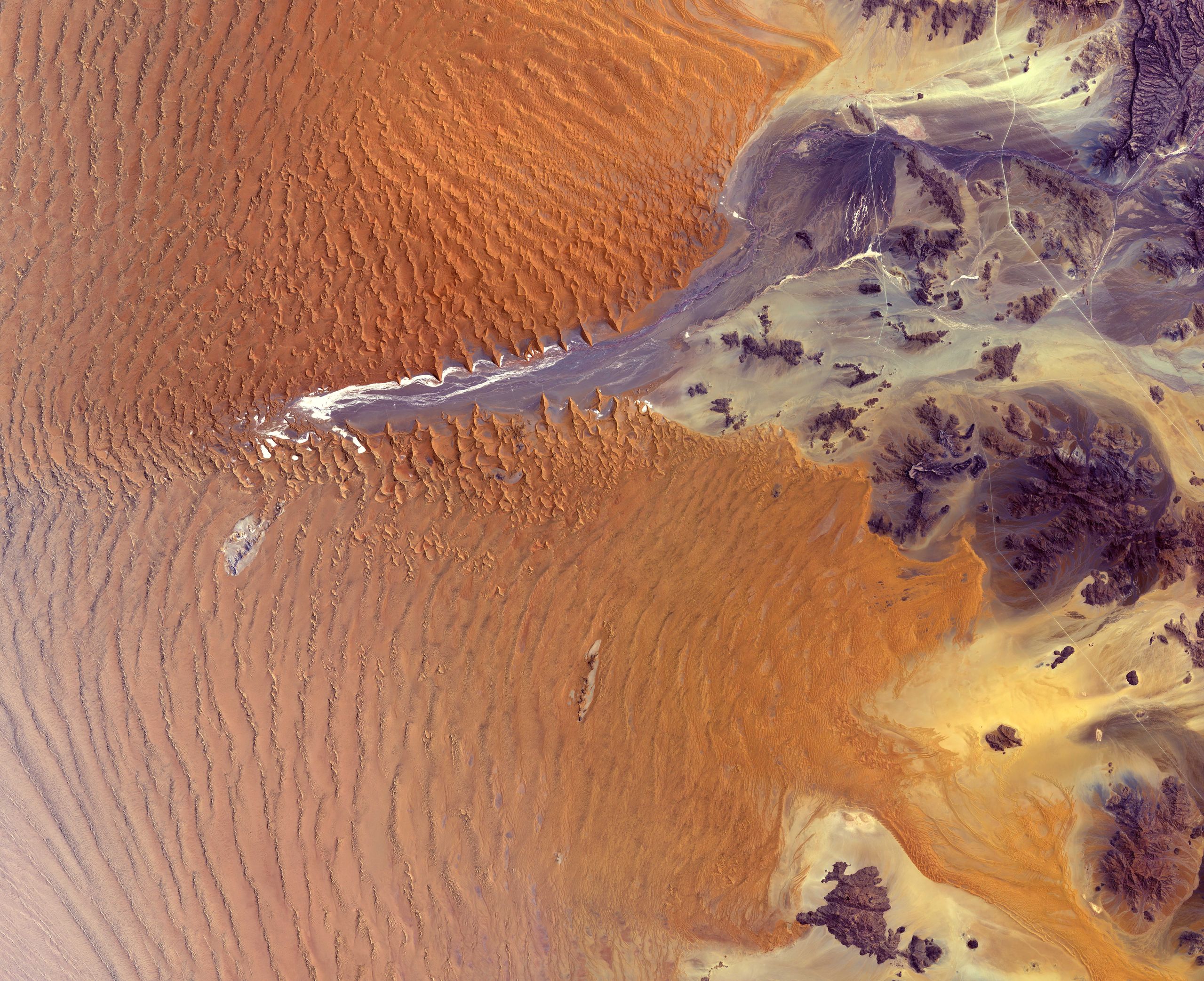This aerial or possibly satellite photograph captures a striking geological landscape characterized by dynamic contrasts in color and texture. The upper portion of the image, predominantly a blend of dark and light oranges, gradually transitions into the lower section where purples become more prominent, especially on the bottom right. The left half of the photograph reveals sand dunes, whose sinuous, wavy lines converge towards the center, giving the impression of wind-sculpted ridges. These dunes appear to be flanked by what looks like a series of rock formations colored in shades of black and dark gray.

As the eye moves from left to right, the sand gives way to what seems to be the remains of bodies of water, now rendered in layers of gray and purple, with the deeper purples suggesting the fluidity of ink spreading across the image. Notably, several areas of the purple expanse exhibit delta-like structures, indicating previous fluvial activity. The interplay of colors and forms is so intricate that a portion of the purple segment even resembles the face of a creature, complete with detailed features like a mouth, dark eye, and black nose. 

This mesmerizing landscape, whether naturally occurring or artistically enhanced, captures a moment of geological and ecological complexity, blending elements of earth, water, and possibly a touch of human interpretation.